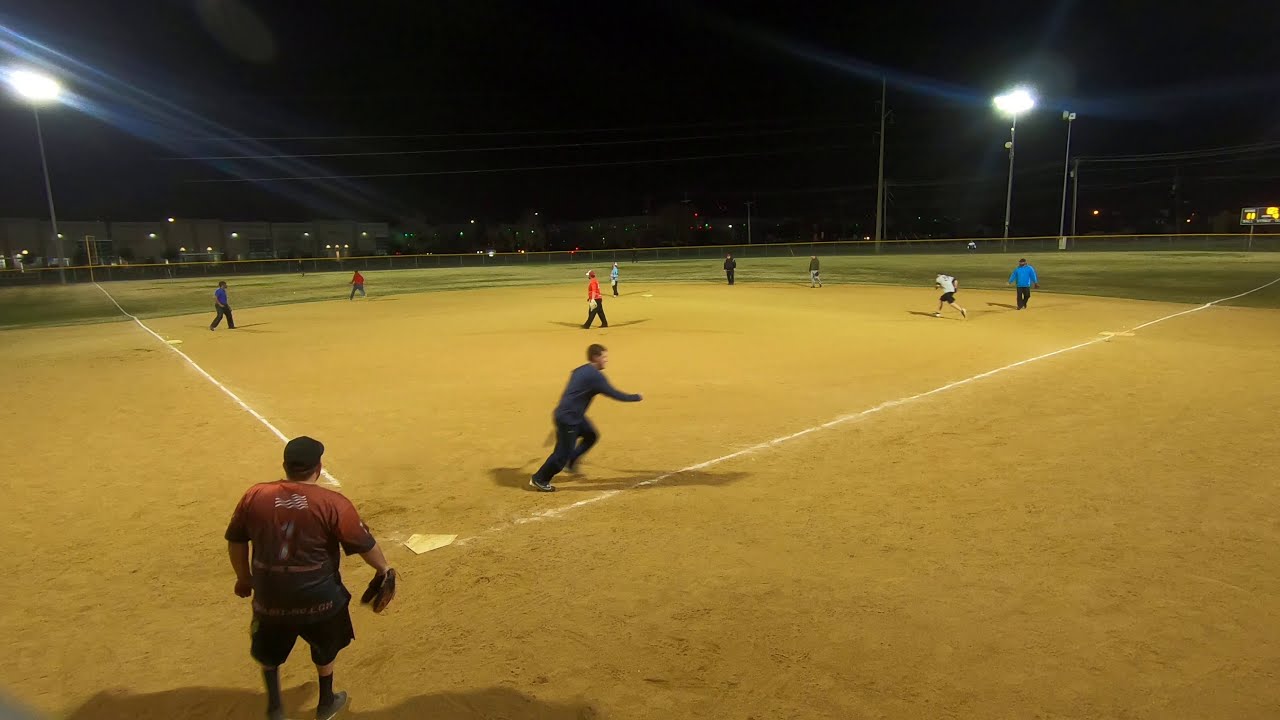The nighttime photograph captures a casual, recreational baseball game set on a field predominantly covered in sandy brown dirt, delineated with white base lines. The outfield is lush with green grass, bordered by a chain-link fence with a yellow top. At the left edge of the field stands a large, mostly darkened white rectangular building, except for a few lights illuminating its adjacent parking lot. The sky above is pitch black, contrasting sharply with the bright stadium lights casting a glow over the scene. Scattered across the field, players dressed in casual, everyday clothing suggest an informal event. Prominently, a heavyset Caucasian man with broad shoulders, wearing a black ball cap, a red shirt emblazoned with the American flag, black shorts, black socks, and gray shoes, stands near the bottom left corner holding a catcher's mitt. He watches as a Caucasian man in a long-sleeved blue shirt and black pants sprints from first to second base. Other players meander around the field casually, adding to the relaxed atmosphere of the game. In the distance, a lit scoreboard punctuates the darkness, contributing to the scene’s quintessentially recreational feel.